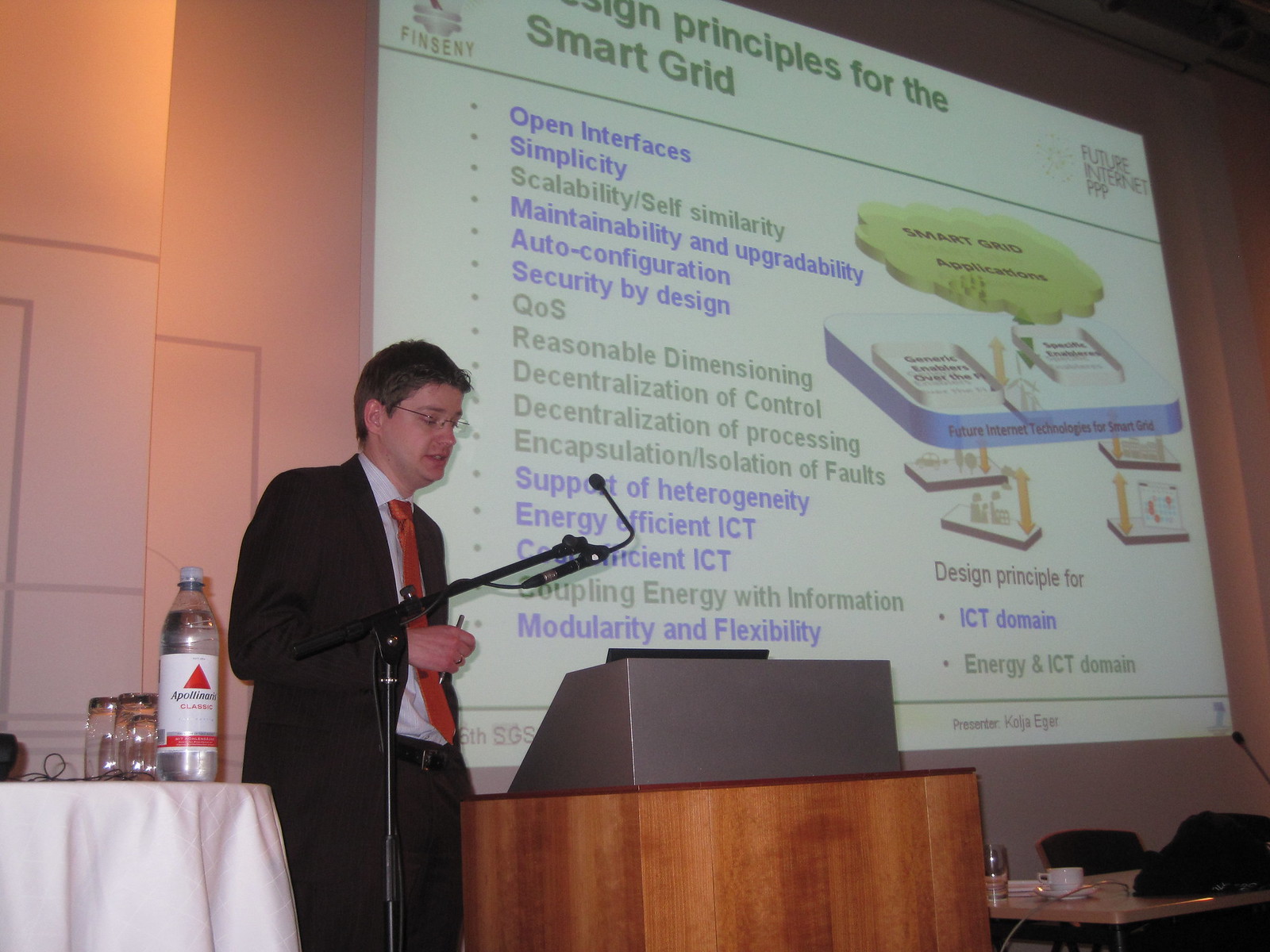In the photograph, a professionally dressed man is giving a speech or presentation, standing behind a gray podium. He is wearing a brown suit with a red tie and glasses, and appears to be around 30 years old. Behind him is a large white projection screen displaying text and diagrams related to "Design Principles for the Smart Grid." The screen lists numerous details including "Open Interface," "Simplicity," "Scalability," "Self-Similarity," "Maintainability and Upgradability," and others, each accompanied by green dots. The text is blue and green, detailing features such as "Security by Design," "Decentralization of Control," and "Energy Efficient ICT." The speaker holds a clicker in his hand, likely to navigate through his presentation slides.

To the left of the speaker, there's a table with a water bottle and glass cups, while to the right, another smaller table with a chair and a teacup suggests that another individual may have been seated there earlier. The backdrop features a pinkish wall with discreet lighting, further indicating a formal, possibly educational or professional event.

Overall, the setting appears to be a modern conference or seminar focused on explaining and extrapolating the principles and methodologies of smart grid technology.